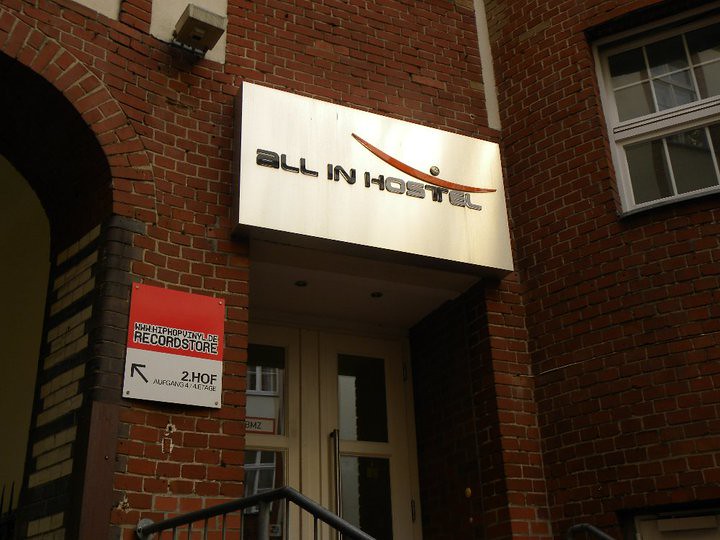The photograph captures a red-brick building from a ground-up perspective, focusing primarily on its front facade. Central to the image is a set of double glass doors, framed in white, and slightly elevated with a black iron railing in front, suggesting the presence of a ramp or steps. Above these doors, there's a silver sign that reads "All In Hostel" in black letters, accented with a red swoosh, serving as the establishment's logo. To the top right of the image, a white-trimmed, multi-pane window is visible. To the left of the doors, an arched brick walkway adds architectural interest. Between the double doors and the arched walkway, a red and white sign points towards a record store, emphasizing the multi-purpose nature of the building. The entire scene is tinged with muted colors and casts a somewhat darker ambiance, indicative of the photo being taken during twilight or early morning hours.